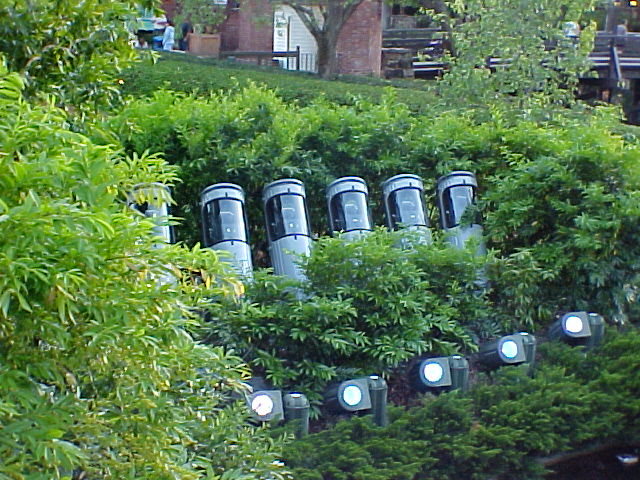This detailed photograph captures a sunny day on the hillside of what seems to be an apartment complex. The hillside, covered in lush greenery, including short, wide bushes filled with vibrant green leaves, creates a picturesque setting. Nestled within the greenery are six unique contraptions or pods, characterized by their upright silver and cylindrical shapes with clear, dark glass windows on the front.

Below these intriguing pods, closer to the foreground, is a row of reflective, half-circle-shaped sensors or solar lights, notable for their bright white centers. These devices are attached to short, vertical black poles that protrude from the ground. The background of the image highlights additional elements of this serene landscape: red brick buildings, a brown fence, and more greenery including trees and bushes. People are visible in the top left corner of the photo, adding a touch of life to the scene. The bright, sunlit sky completes this vibrant and dynamic outdoor environment.